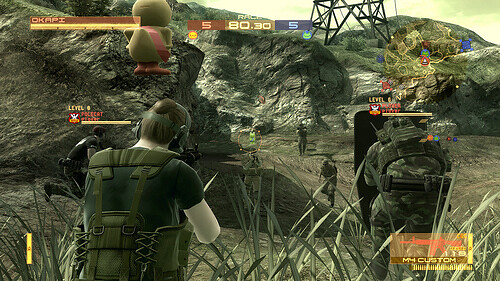This detailed caption describes a screenshot from a video game, depicting a multiplayer-style mode in action. At the top of the screen, a timer reads "80:30" underneath the word "RACE." Both the left and right corners of the top section display a red block and a blue block, each showing the number "5." 

In the upper left-hand corner, a red box contains a yellow line representing a health bar with the text "OH COPY OKAY API" beside it. Yellow health bars are visible above two characters, positioned to the left and right, who are clad in military-style outfits and appear to be engaged in combat.

A green and yellow mini-map is located in the upper section. The bottom right corner features a yellow block displaying "M4 CUSTOM 118" along with a red image of a rifle. Additionally, the upper left corner includes an image of a duck with a red banner and orange feet, suggesting a possible connection to a Metal Gear game, potentially "Metal Gear Survive," based on the familiar user interface design.